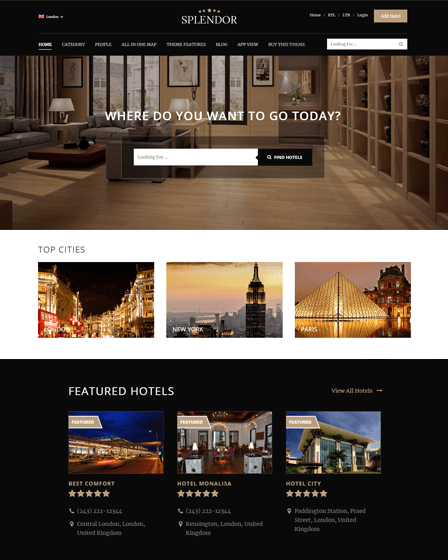**Caption:**

This screenshot captures an unknown web page design centered around a travel or accommodation theme. At the top, a black banner features the word "Splendor" in elegant white letters, flanked by five curved stars above it. Directly beneath is a blurred menu bar comprising options like Home, Category, People, All-in-One Map, Theme, Blog, and App View, accompanied by a search bar.

The main content begins with a photograph of a stylish living room showcasing wooden floors and dark tan walls. On the far right is a wooden shelving area, while the far left features a gray seating arrangement around a low dark brown coffee table. Large windows on the back wall allow a view of neighboring houses.

Below this photo, the text "Where do you want to go today?" appears alongside a search bar inviting users to look for hotels. Under the banner "Top Cities," three iconic cityscapes are displayed: a night view of London, the New York skyline, and the Louvre Pyramid in Paris.

Further down, a black section highlights featured hotels with a prompt to "View All Hotels." It lists several top-rated accommodations, including 'Best Comfort' with five stars, 'Hotel Mona Lisa' with five stars, and 'Hotel City' with five stars, though the descriptive content under each is too blurry to decipher.